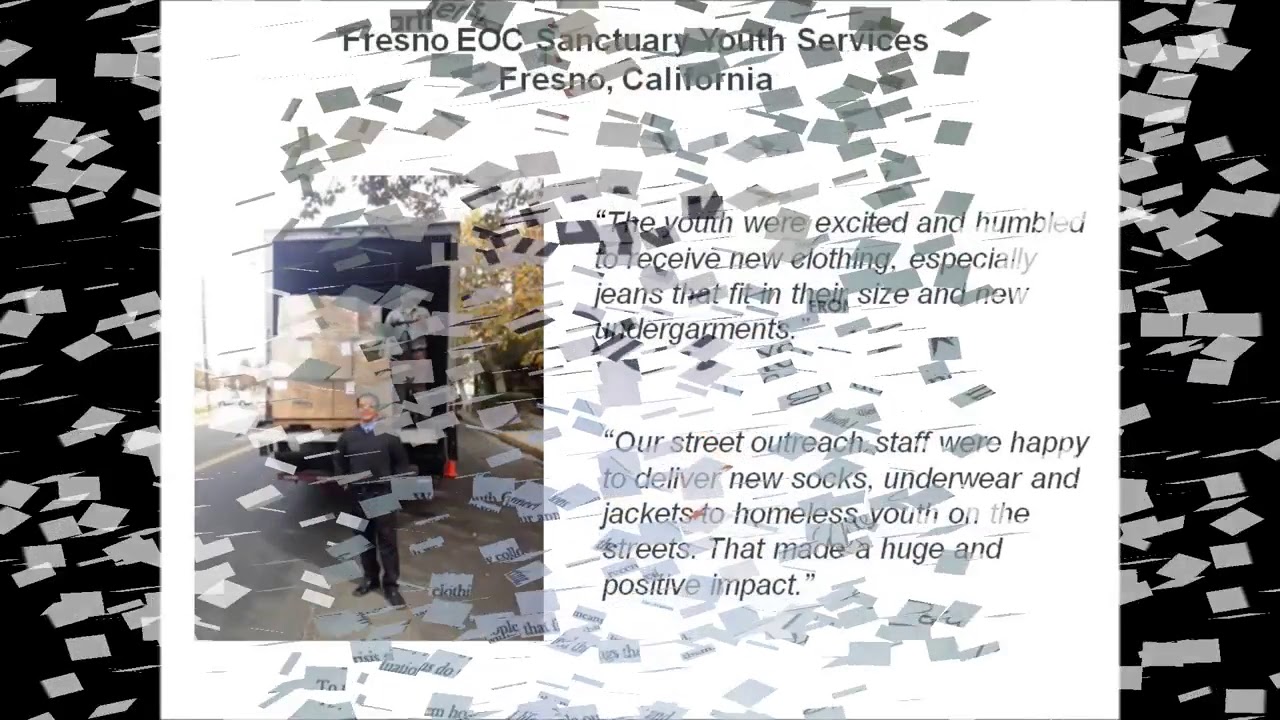The image showcases a graphic for Fresno EOC Sanctuary Youth Services, Fresno, California. Central to the image is a white box with black text detailing a heartfelt message: "The youth were excited and humbled to receive new clothing, especially jeans that fit in their size, and new undergarments. Our street outreach staff were happy to deliver new socks, underwear, and jackets to homeless youth on the streets. That made a huge and positive impact." Adjacent to this text, on the left, is a photograph depicting a man dressed in black attire standing in front of an open truck filled with cardboard boxes, parked on a street. The entire image is overlaid with a unique texture resembling scattered, bit-ripped pieces of paper, giving the impression of confetti raining down. This effect extends even to the black borders framing the left and right sides, evoking a sense of motion and dynamic composition. This visual narrative combines the textual message of compassion and impact with an artistic overlay, creating an engaging and poignant portrayal of community service.